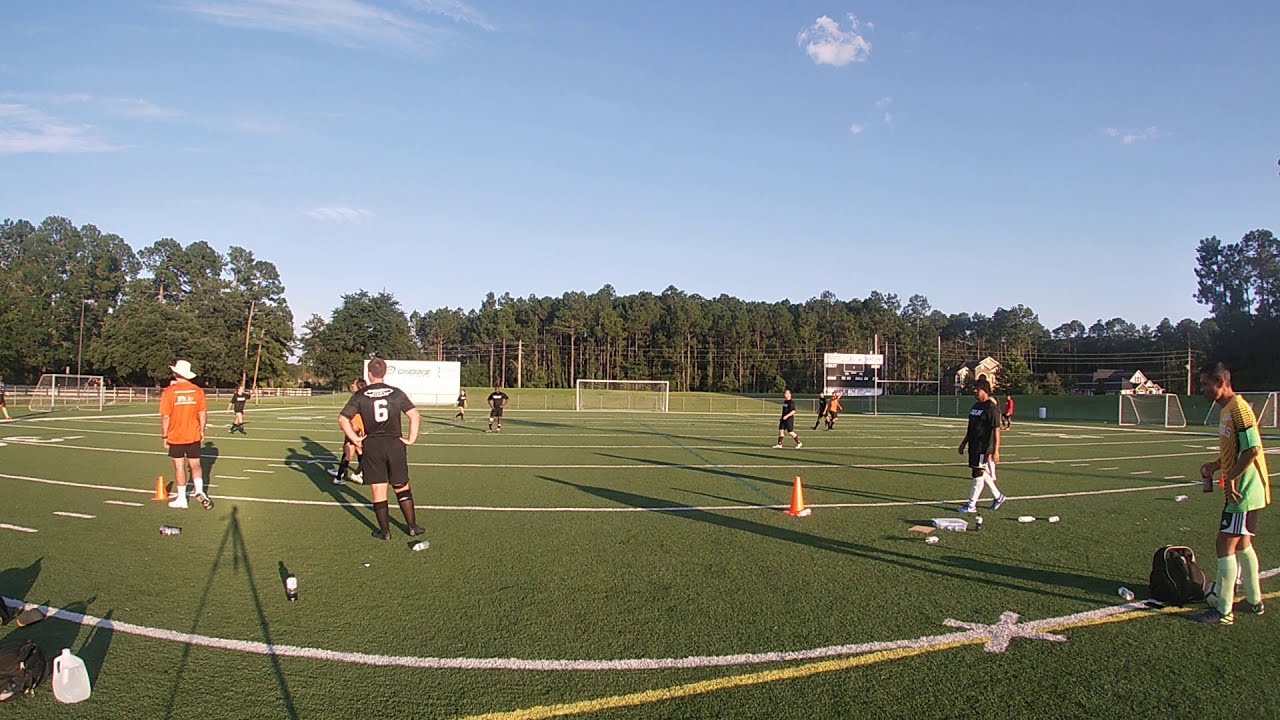The photograph captures a sunny scene at a soccer practice session on a well-maintained field marked with white and yellow lines, possibly doubling as a football field. A blue sky with scattered wispy clouds stretches above a dense backdrop of green trees encircling the field. Scattered across the green turf are twelve individuals clad mainly in black jerseys, black shorts, and long black socks, characteristic of standard soccer gear. One particular player, positioned on the left, has the number 6 in white on his jersey and stands with his hands on his hips, gazing into the distance. Nearby, another person in an orange t-shirt, white floppy hat, white socks, and dark shorts also looks into the field. To the far right, partially blocked by the number 6 player, stands someone, possibly an equipment person, next to a gear bag and an orange traffic cone. The field features multiple soccer goals, three in total, positioned in the far distance and on either side. A green fence surrounds the area with a scoreboard visible towards the center, all under a late-day sun casting long shadows.